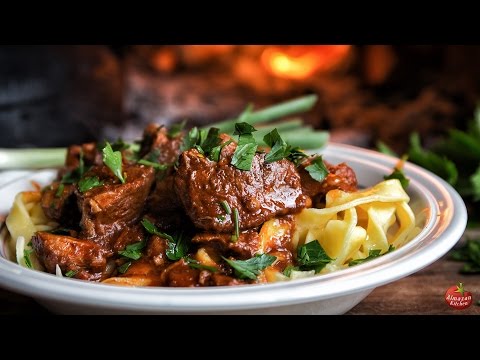The image captures a beautifully presented dish featuring a round, white plate with a raised rim, filled with yellow noodles topped with shiny, seared braised beef. The beef, possibly a short rib or steak, is glazed and scattered with fresh green cilantro or herbs, adding vibrant color to the dish. The focus is sharply on the food, with the background artistically blurred, hinting at a cozy fireplace or campfire ambiance. The setting includes additional greenery on a brown table, contributing to the rustic and inviting atmosphere. Notably, the bottom right corner features a logo emblazoned on a tomato, suggesting the image might be part of a food advertisement. The overall composition is enhanced by the soft glow of the fire in the backdrop, creating a warm and appetizing visual.